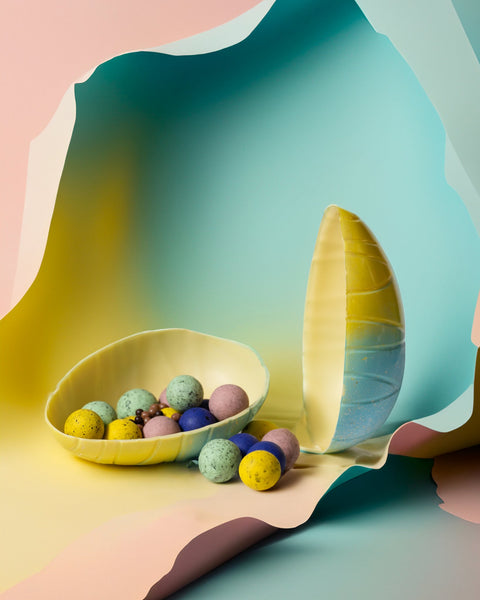This vertically-aligned rectangular image depicts a plastic egg that has been cracked open along its edge, revealing an array of small, marbled, colored balls inside. The broken egg is positioned on crinkled, multi-colored paper. The egg's bottom half, resting centrally, is filled with these balls, which resemble Whopper candy with speckles. The balls are primarily teal, yellow, pinkish-purple, and blue, with darker spots. Some balls have spilled out and rest on the paper. The egg's top half, blue at the bottom and yellow at the top, stands vertically to the right. The background paper is a blend of colors—blue on top, yellow on the left, and pink on the right, creating a vibrant and visually engaging scene. The interior of the egg is a light, smooth tan, providing a stark contrast to the colorful exterior and contents.